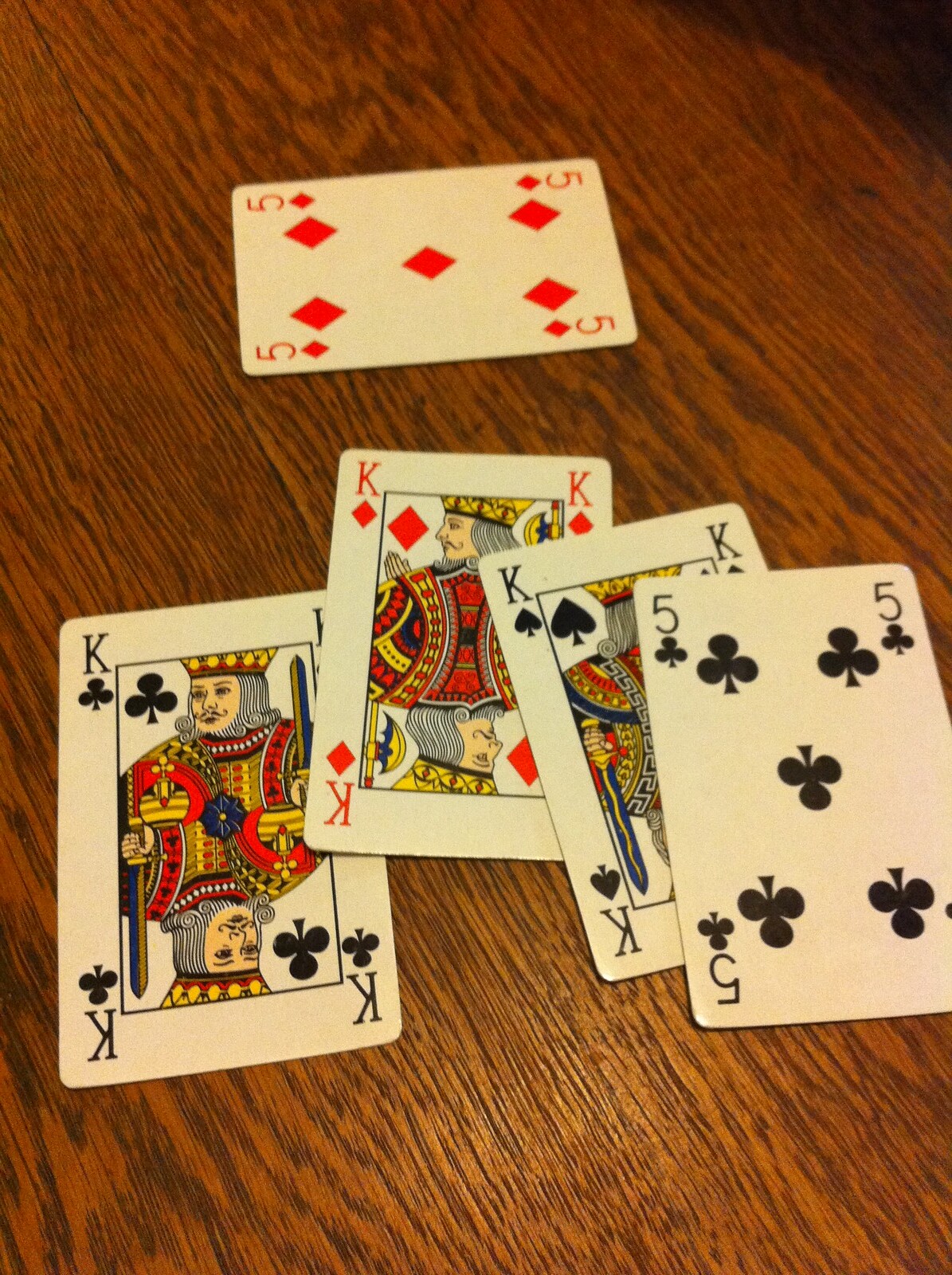A detailed close-up photo showcases a wooden table with a noticeable grainy texture. The table's wood features a light brown base accented with dark brown, almost black, markings that highlight the natural granules. Splayed across the table horizontally, four playing cards overlap each other in a visually engaging arrangement. From left to right, the cards are the black King of Clubs, the red King of Diamonds, the black King of Spades, and the black Five of Clubs. Above these cards, oriented in the opposite direction and lying horizontally, is a solitary red Five of Diamonds. This card stands alone, unaccompanied by any other cards nearby. In the upper right corner of the image, a dark shadow looms, suggesting the presence of an unseen person casting it.